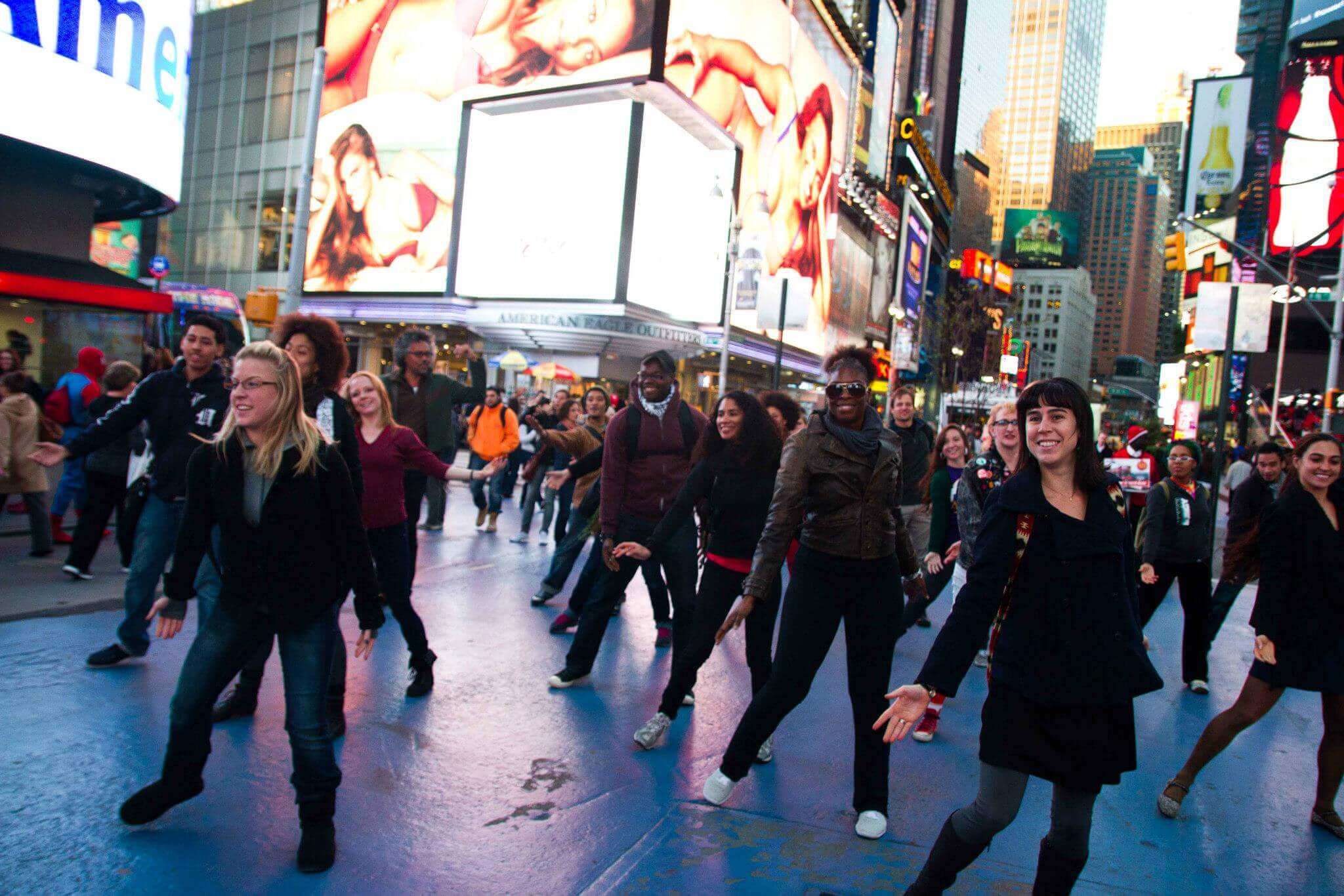In this striking image of Times Square in Midtown Manhattan, a lively flash mob takes center stage amidst the backdrop of iconic skyscrapers and dazzling electronic billboards. Around 30 to dozens of individuals can be seen dancing in unison, their coordinated movements creating a dynamic and joyful atmosphere. Participants, dressed in winter jackets indicative of late autumn or early winter, are spaced out evenly across the shiny, wet pavement, which reflects the myriad of city lights. Prominent advertisements, including a Coca-Cola sign and lingerie ads featuring celebrity models, frame the scene, affirming the location as the bustling epicenter of New York City. The dancers, many smiling and engaging with the camera, are captured in mid-action, some kneeling or extending their arms, evoking the spirited spontaneity of an old-school flash mob. This captivating snapshot captures not only the energy of the dancers but also the vibrant essence of Times Square, making it a quintessential New York moment.